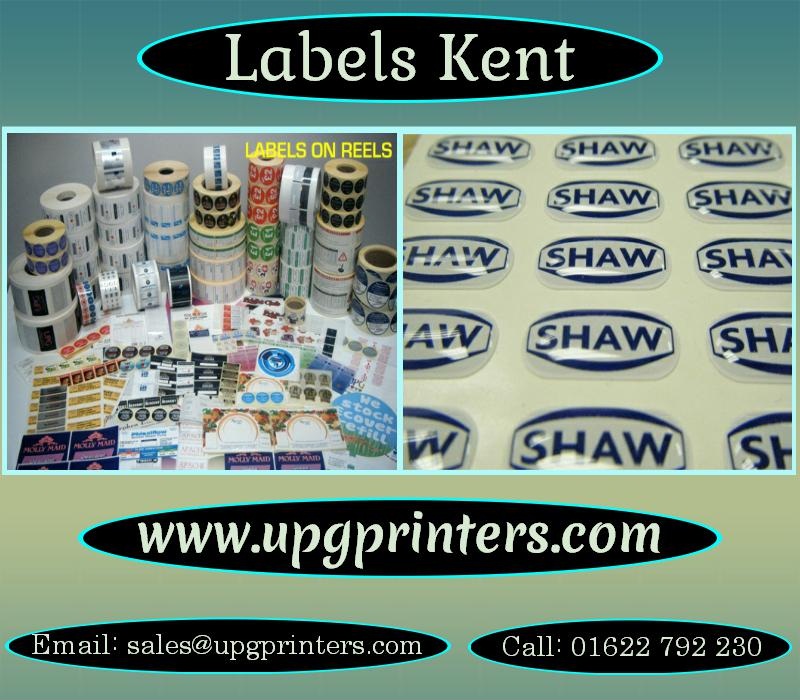The image is an advertisement featuring two photographs side by side. The left photograph displays a white desk with a variety of label reels, and in the background, stacks of label rolls are visible. At the top of the left photograph, there is a black oval shape with a light blue border that contains the text "Labels Kent" in white. Below this, additional black ovals contain the text "www.upgprinters.com" on the left, "email: sales@upgprinters.com" in the middle, and "tel: 01622-792230" on the right.

The right photograph has an ivory-colored background with the word "Shaw" repetitively printed in blue letters across the entire background. These letters are arranged in multiple rows, creating a grid pattern. The advertisement prominently features the company's website, email address, and phone number at the bottom, tying both images together as part of the company's promotional material.